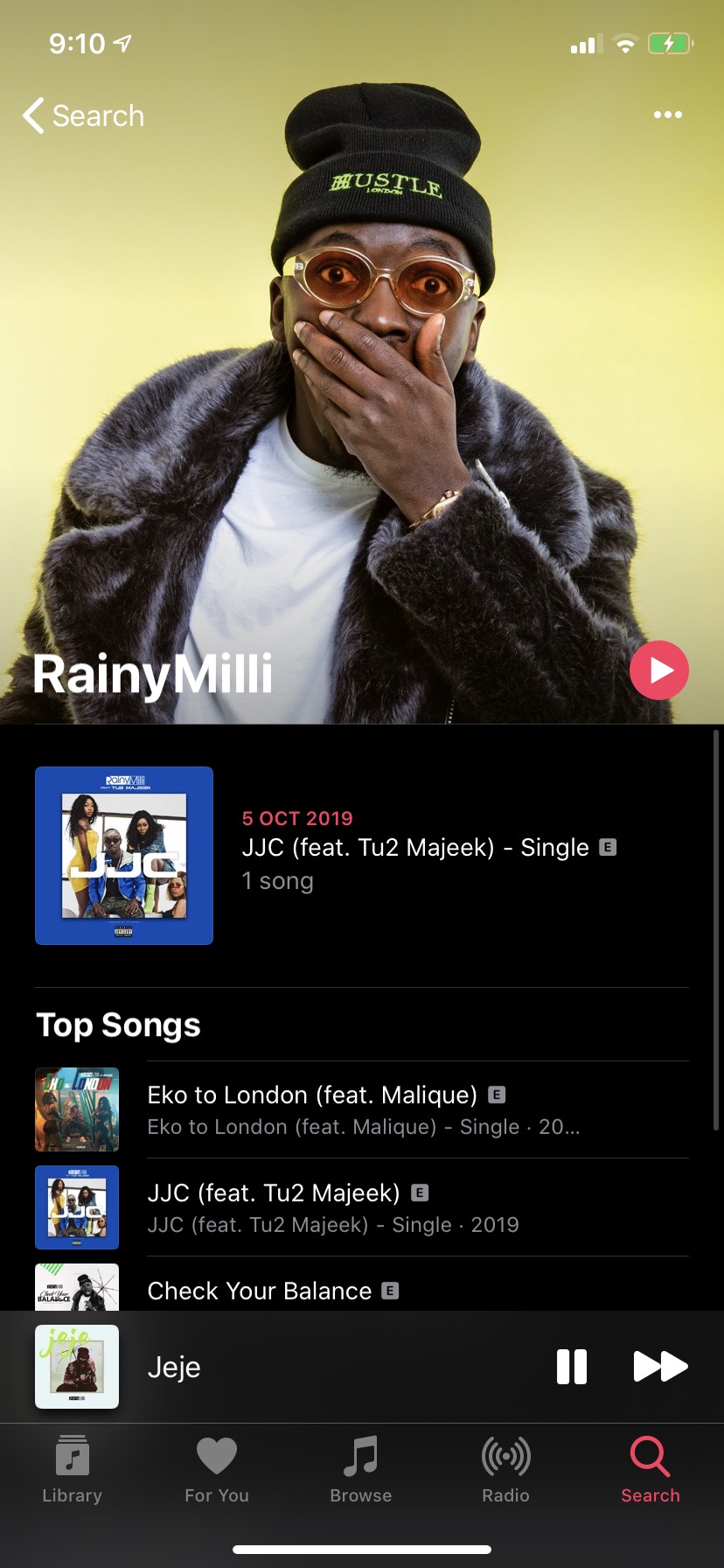This image captures the screen of a cell phone at 9:10 AM, indicated by the time displayed in the top left corner. The top right corner features icons for cellular connection, wireless signal, and a battery that is charging. Directly below this is a small arrow pointing to the left with the word "Search" beside it. On the far right are three small white dots arranged vertically.

The main image showcases an African-American man, seemingly middle-aged, looking directly at the camera. He is wearing a black stocking cap with the word "Hustle"—although the 'H' may be stylized or different—prominently displayed in the front. Below this, in smaller text, the word "London" is visible. The man sports glasses that resemble goggles, with his eyes wide open. His left hand is covering the lower part of his face. He is adorned in a fur coat over a white t-shirt, the sleeve length of which is not clear. A watch is just barely visible from under the cuff on his right arm.

At the bottom of the picture, the text "Rainy Millie" is displayed, along with a play button situated on the far right. Beneath this is an album cover featuring the text "Rainy Millie," and "JJC." The album cover shows a man flanked by three women. It includes textual details: "5 October 2019, JJC featuring 2 2 Majik, single, one song." Below this, the section labeled "Top Songs" lists tracks including "Eco to London featuring Malik, JJC featuring 2 2 Majik," "Check Your Balance," and "JJC," each associated with their respective album or song covers.